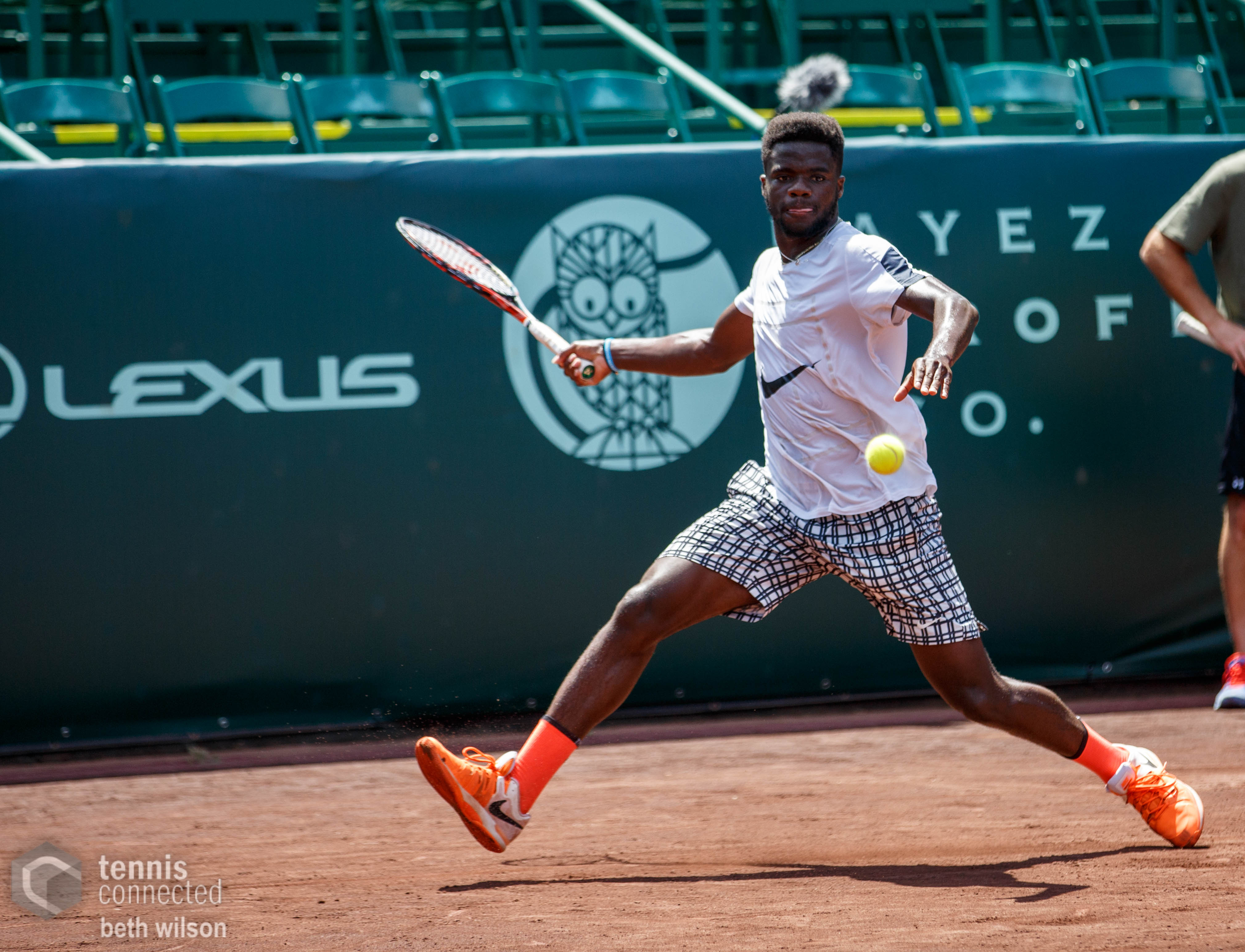This photograph captures tennis player Franklin Tiafoe in mid-action as he prepares to hit a hovering yellow tennis ball. Tiafoe is sporting a white Nike t-shirt emblazoned with the Nike logo at the center, paired with distinctive white shorts featuring a black plaid pattern of vertical and horizontal lines. His vibrant orange socks with a black stripe at the top, along with his orange and white Nike tennis shoes, add a splash of color to his attire. Tiafoe is in motion, running with his right hand, which is holding an orange and black tennis racket, poised for a powerful swing. The intense focus on his face is evident, possibly indicated by the concentrated position of his mouth. The background reveals the stadium stands, with banners of sponsors such as Lexus adorning the lower section. Distinctively at the bottom left corner, the text "Tennis Connected, Beth Wilson" is overlaid, crediting the photographer and publication.